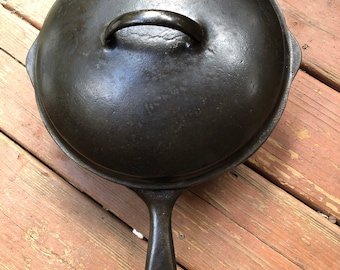The image features a color photograph of a cast iron skillet with a domed, dark metallic lid, situated on a light to medium brown wooden surface that appears to be an old picnic table or wooden deck with visible scratches, chips, and peeling paint. The skillet is centrally placed, but the close-up, square framing cuts off part of the handle and the top portion of the pan. The lid has a raised handle at the center, and a reflective light highlights its metallic surface. The composition focuses solely on the skillet and the worn wooden background, with no people or text present.